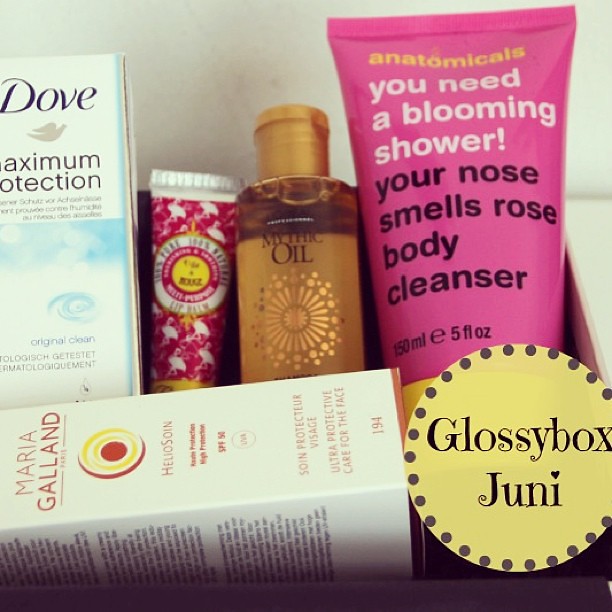The image is a large square depicting a curated selection of self-care and beauty products neatly arranged inside a box. On the right side of the image, the straight white edge with a purple interior marks the boundary of the box. In the upper left-hand corner, there is a box of Dove Maximum Protection deodorant. To its right, there's a small, blurry container of lotion that is pink and white with a yellow cap. Further right, there's a brown and gold snap-top bottle labeled Mythic Oil. Next in line is a dark pink tube of lotion with bold yellow letters that read "anatomicals" followed by "you need a blooming shower" in white, and in black text, "your nose smells rose body cleanser." Just beneath these, a white box labeled "Maria Galland" with some additional text in French is positioned perpendicular to the other items. In the lower right-hand corner of the image is an overlaid circular logo featuring light brown with dark brown dots around its perimeter, and inside it bears the black text "glossybox" with "JUNI" beneath it. This arrangement suggests the products are part of a beauty and skincare subscription box, highlighting the variety of items from brands like Dove, Mythic Oil, and Anatomicals.